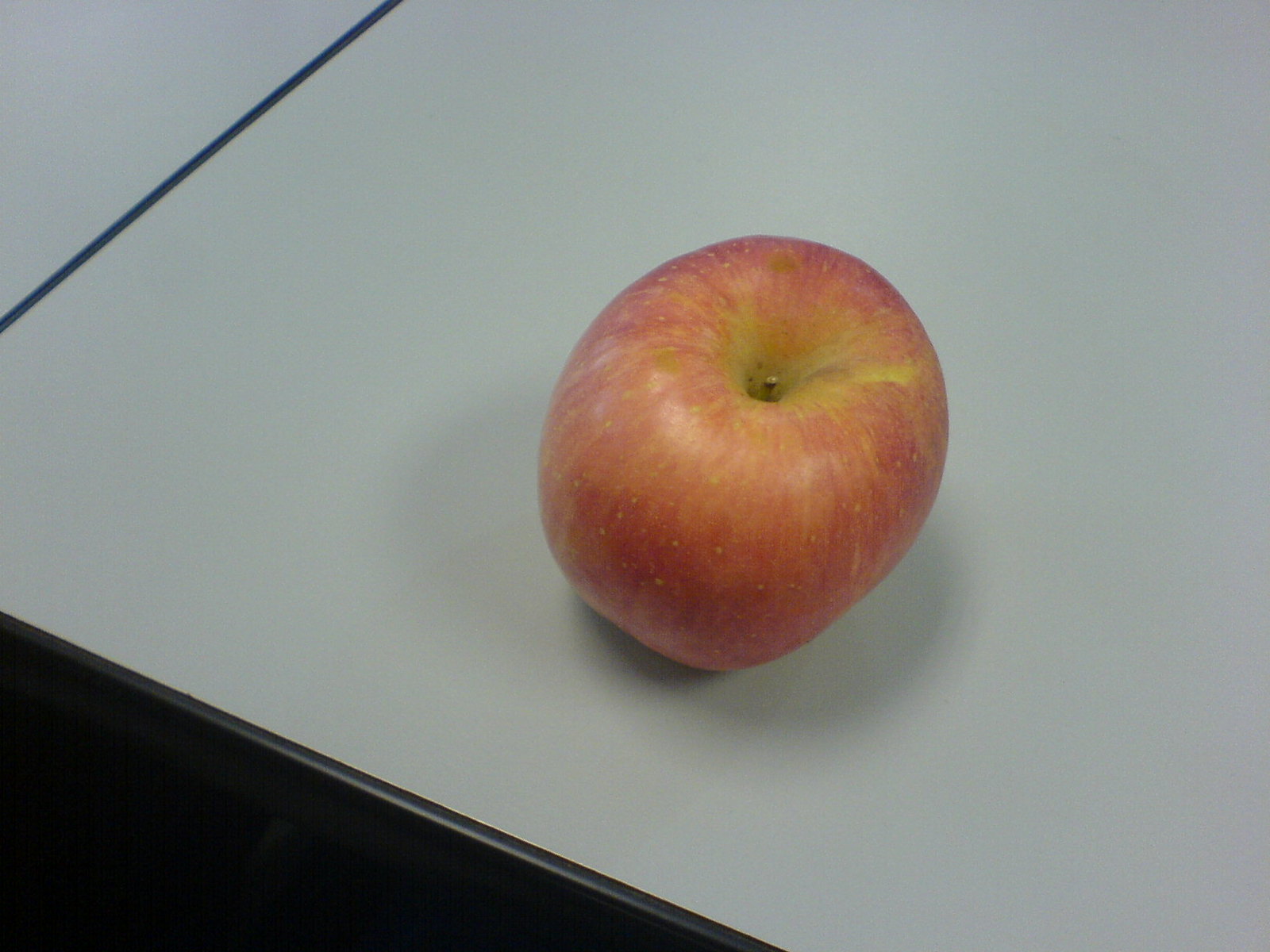A photograph captures a single apple resting on a white table with a black rubber edging. The table appears to either be adjacent to a similar table or one that splits and reconnects, indicated by a visible central seam. The camera angle is slightly off to the side, revealing the table rim in the bottom left corner and leaving dark space below. The apple itself is predominantly red with a mixture of orange and yellow hues, suggesting it's mid-transition to full ripeness. A short stem is still attached, sprouting from a yellow patch near the top. The apple's variegated coloring hints at its sweet flavor, making it a likely lunch table companion.